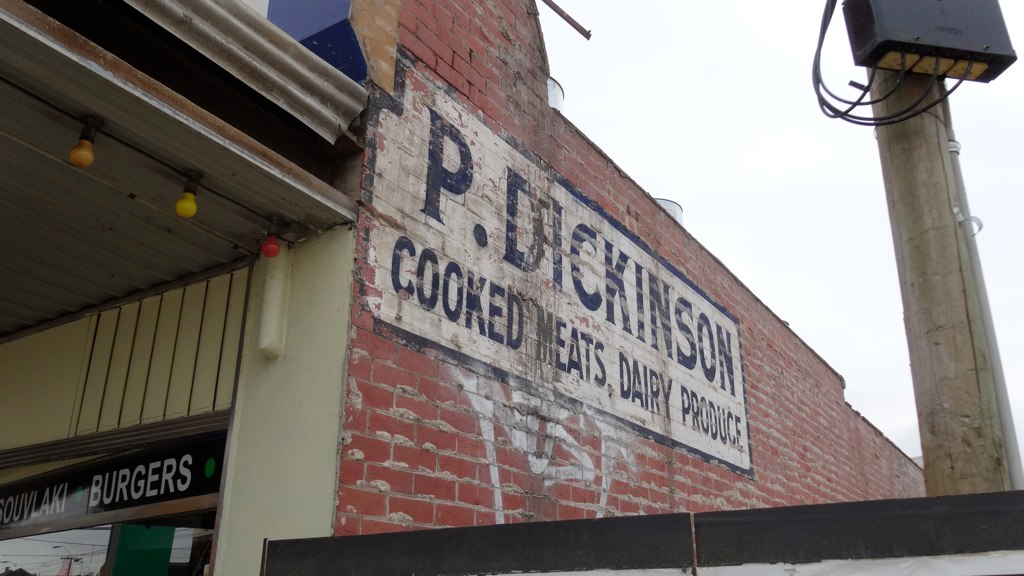The image is a photograph taken from the ground looking up on an overcast day, capturing an old, worn-out red brick building. Prominently displayed on the side of the building is a weathered white painted sign bordered with blue or black, reading "P. Dickinson Cooked Meats Dairy Produce," hinting at this building's historical past. The sign shows signs of aging and possible graffiti. Adjacent to this section of the building is a small storefront with beige walls and a tin awning adorned with brightly colored bulbs in red, yellow, and orange. Visible near the awning are parts of advertisements, including the partially visible word "souvlaki" and "burgers" in white text on a green background. In front of the building runs a steel fence or gate, and a large telephone pole with wires and a black box is situated to the right. The photograph's angled perspective accentuates the aged and somewhat gritty atmosphere, with no people visible in the image, lending it a desolate and historical feel.